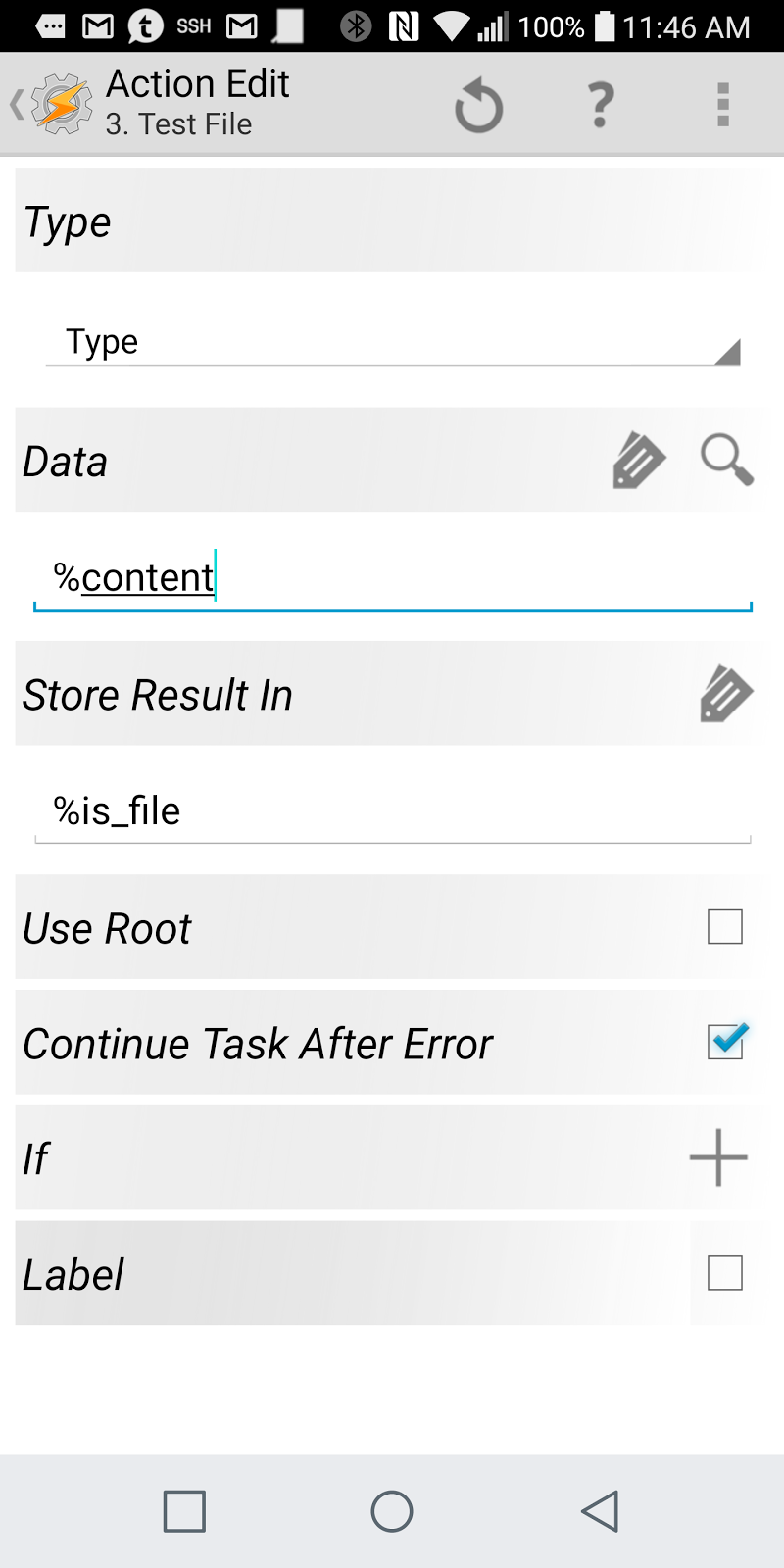A screenshot taken from a smartphone. 

At the top, there's a thin black border. From the left to the right, there's a small tab with a tip pointing left, three black dots in the center, followed by a white square containing a black "M," white top with black "T," then "SSH" in white, followed by a black square with another "M." Adjacent to these elements is a large, blank white rectangle. The icons above indicate Bluetooth is off, a square with an "N" in it, full Wi-Fi signal (4 out of 5 bars), 100% battery charge, and the time displayed is 11:46 a.m.

Beneath this section, approximately an inch below, there's a gray tab. On the left side of this tab, there's a settings icon with a yellow lightning bolt. To its right, it says "Action Edit" in black text, and below that text, "Three Point Test File." Over on the right is a refresh button, followed by three gray squares.

Moving further down, there's another gray bar labeled "Type," with a white or gray line labeled "Type" underneath it. Beneath that, there's a gray rectangle labeled "Data," followed by a blue line with "Content" above it. Continuing down, there's another gray rectangle labeled "Store Results In," followed by a text box with "Percentages File." 

There are four additional gray rectangles in a row with the following labels: "Use Root," "Continue Task After Error," "If," and "Excellent Label."

At the very bottom, there's a gray bar with a darker gray square, a darker gray circle in the center, and a sideways triangle pointing to the left.